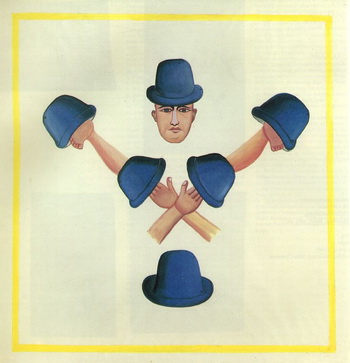This detailed artwork features a cartoony and symbolic image framed by a bright yellow border on a pale yellow, almost transparent background, faintly displaying what seems like newspaper articles. At the center of this square painting floats the stoic, clean-shaven face of a man wearing a navy blue bowler hat. Below his head, two hands crisscross, each holding a blue bowler hat. Further down, legs extend from these hats, each wearing another blue hat perched on bare feet. At the very bottom of the composition sits a singular blue bowler hat. The juxtaposition of these elements creates a visually intriguing, almost surreal portrayal, as if forming a symbolic structure that is both whimsical and mysterious.